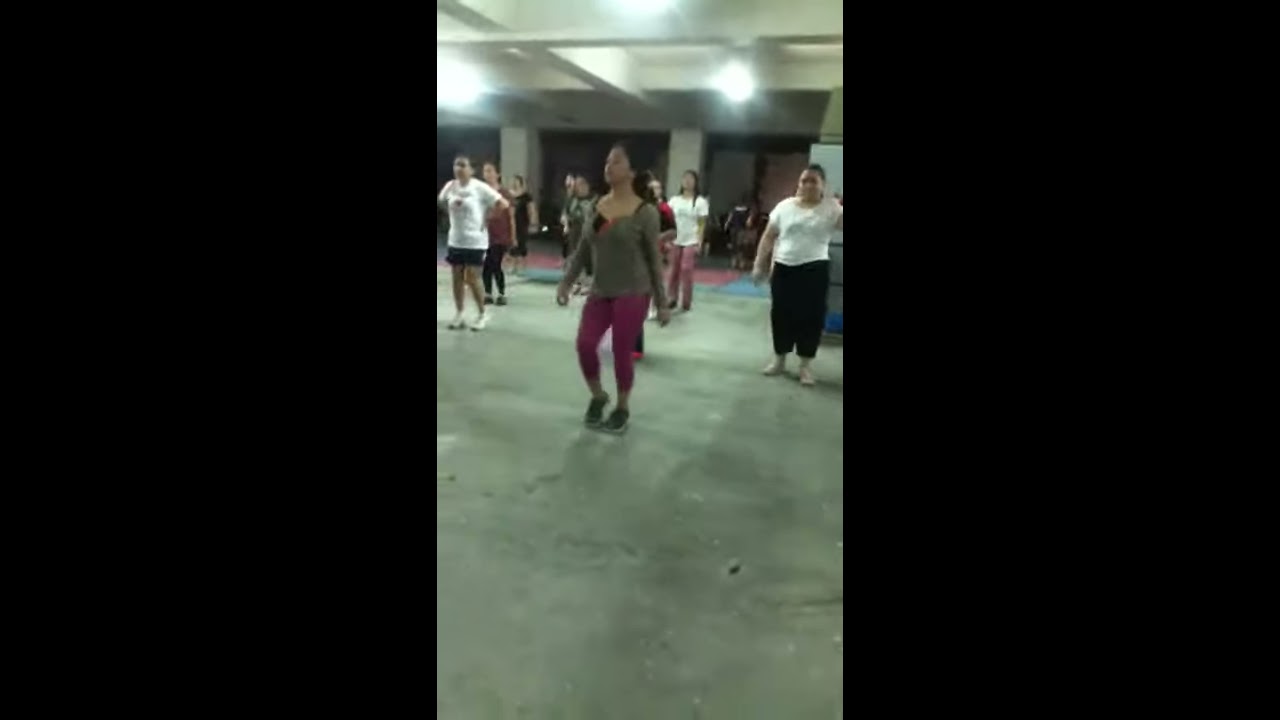In the center of this horizontally-aligned rectangular image, enclosed by large black borders on the left and right sides, stands a vertically-oriented picture depicting a diverse group of women in an exercise class. The scene is set indoors on a concrete floor, beneath a white ceiling with visible beams and bright spotlights highlighting the space. The group appears to be following a workout routine, possibly a fitness or Zumba class.

Central to the image is a woman with long black hair, wearing a long-sleeve athletic top and purple leggings, along with tennis shoes. She is positioned at the forefront of the group, her arms extended to her sides in a poised stance. Flanking her, a woman on her right sports black sweatpants and a white t-shirt, while another on her left wears black shorts and a white t-shirt. Behind and around the central figure, approximately 15 people stretch into several rows, though only those in front are distinctly visible against the possibly blurred background, with hints of red and blue exercise mats.

The participants, all dressed in various athletic attire, are uniformly facing one direction, suggesting synchronized movements and collective engagement in their fitness activity.